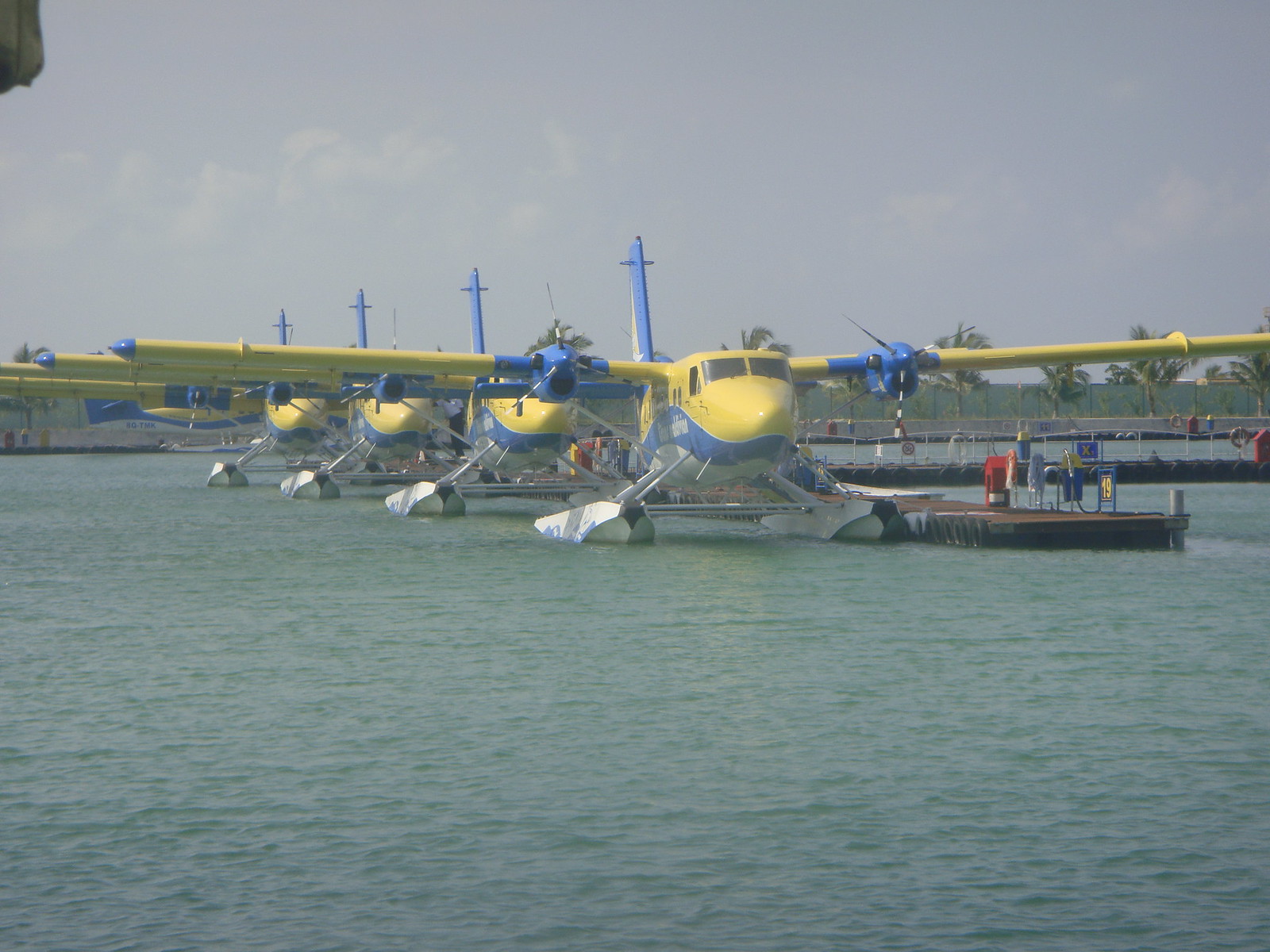The image depicts a well-lit, outdoor scene of a serene bay with a collection of seaplanes moored alongside a dock. The water in the foreground appears calm with a bluish-gray or light green-blue tint, and the clear sky above is adorned with a few white clouds. The photograph, taken from a slightly diagonal front view, highlights a row of seaplanes lined up one after another, extending into the background.

Each seaplane features a predominantly yellow body with blue elements, including blue propellers, a blue tail accented with white, and blue detailing on the wings and nose. Some planes also have a blue stripe running along the fuselage. The seaplanes rest on floats in the water, giving them a blocky appearance due to the structure supporting their landing gear.

In addition to the seaplanes, the image also shows the dock running along the right side and to the center, strewn with various details such as gasoline pumps and tanks. The dock appears brown with some red and blue elements. In the distance, palm trees are visible, adding a touch of tropical scenery to the background. The image is crisp, well-composed, and captures the tranquility of this aquatic setting with great detail and clarity.